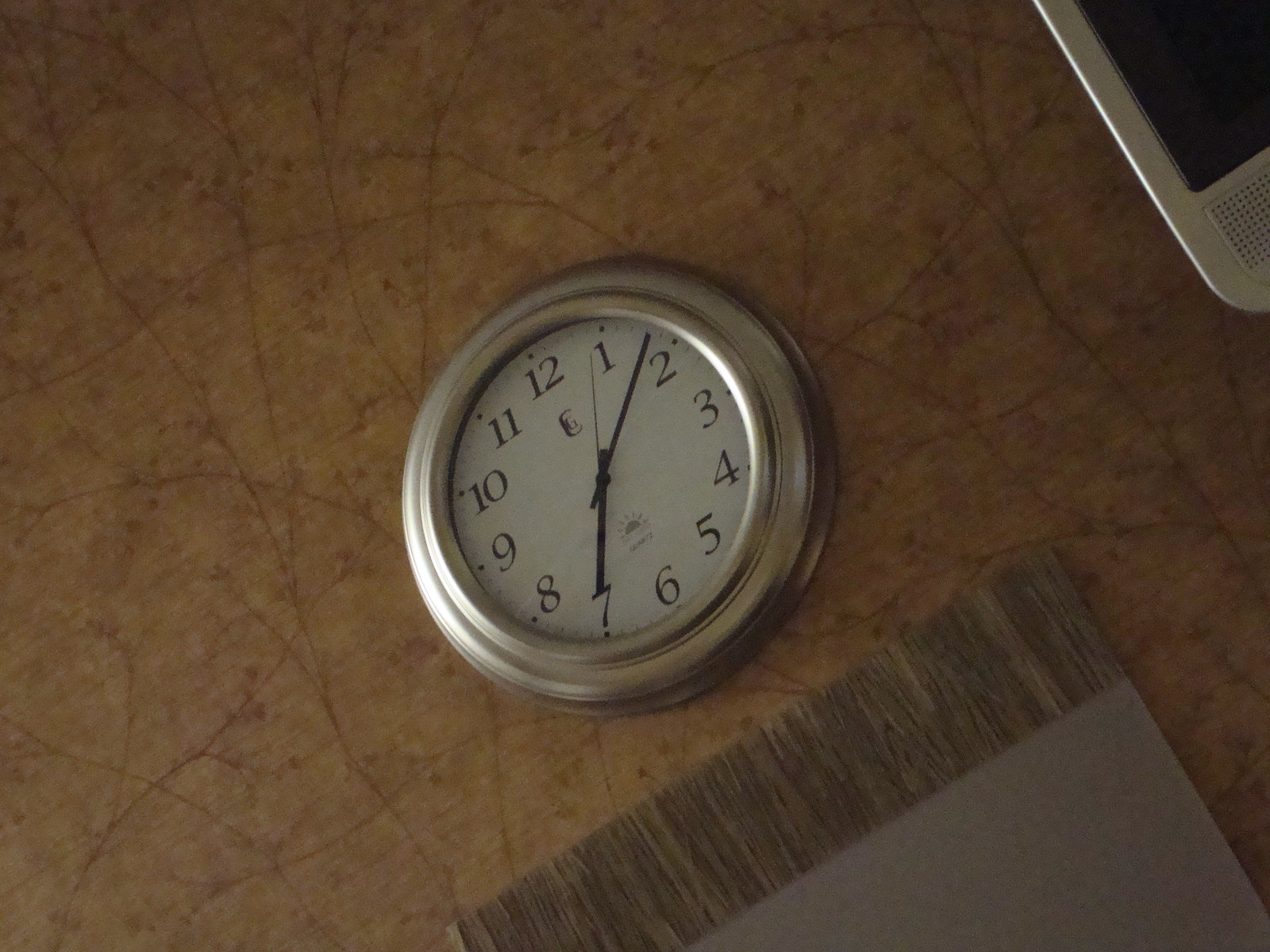This image, a realistic photograph, captures a detailed scene with various elements. The background is either a floor or a wall with a tan beige-colored surface, adorned with darker brown lines resembling twigs and tiny buds, creating a patterned effect. In the lower right, a dark blue rug with tassels extends towards the upper left, likely indicating that the setting is on the ground. A prominent feature is an analog clock positioned centrally in the frame. The clock has a silver or stainless steel edge, with a white face and black numbers from 1 to 12, each with a black dot above. The hour hand is at 7, the minute hand is between the 1 and 2, and the second hand points at 1. The clock face includes a C with a G inside at the 12, and a light gray half-sun decal above the 6. Additionally, a quarter of a tablet is visible in the upper right corner, partially cut off by the image's edge. The scene also includes some sort of brown table runner with tassels or a similar object below the clock. Overall, the composition captures various textures and details, creating an intricate and engaging image.